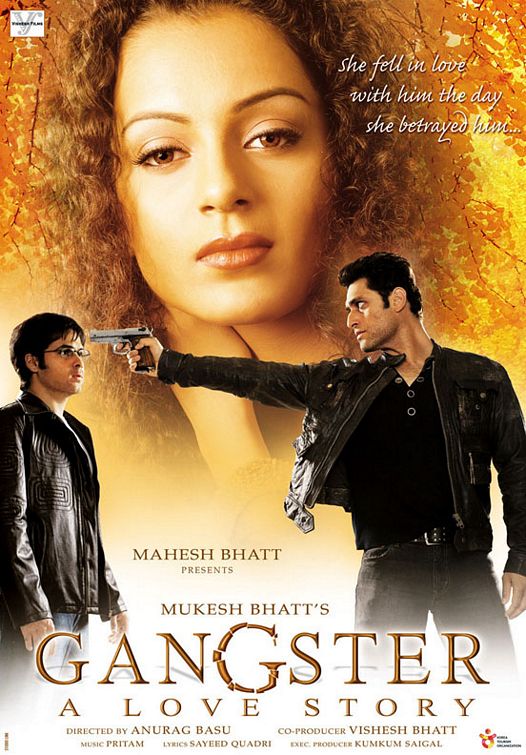The image is a vertically oriented movie poster with a golden yellow and white color scheme. Dominating the background is a large close-up of a woman with European features, brown curly hair, vivid red lips, and a serious expression. Fall-colored trees and leaves surround her hairline, adding a seasonal touch. In the foreground, two men in black leather jackets engage in a tense standoff. The man on the right, bigger and older, has short black hair and is clean-shaven. He holds a gun with a brown handle and a stainless steel barrel pointed at the forehead of the smaller man, who also has short black hair, wears glasses, and looks fearful. The text at the top of the poster in white script reads, "She fell in love with him the day she betrayed him." The bottom of the poster features gold font on a white background displaying the title "Gangster, A Love Story." The director's name, Mukesh Bhatt, appears prominently above the word "presents," with additional details about the actors and crew in small print below.